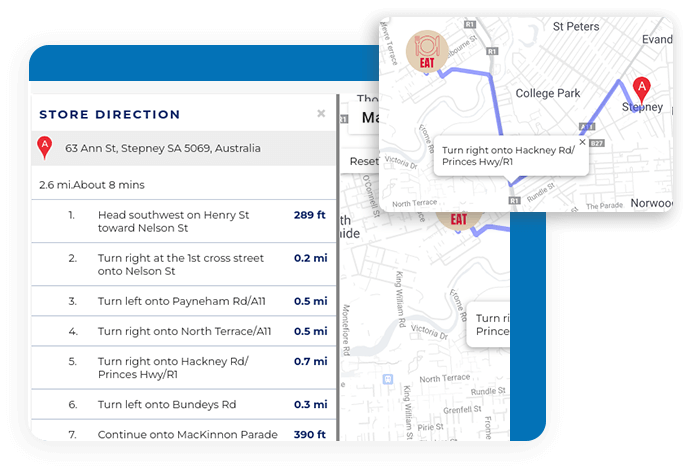The image features a detailed screenshot from a GPS navigation app, possibly Google Maps, showing step-by-step directions to a restaurant. The visual is divided into two sections. The left section, which is larger and highlighted with a blue background, lists the directions in a numbered sequence from 1 to 7. These directions begin at 67 Stephanie's S.A. Street, Australia, and provide incremental steps such as heading southwest for 289 feet, followed by various turns and distances, culminating in a final instruction to turn left onto Bundy's Road and then continue onto McKinnon Parade, covering a total distance of 0.3 miles in the final steps.

The right section of the image displays an enlarged map, emphasizing the route visually. This map starts at Stephanie's Street, with the path clearly marked in blue, leading to the restaurant, which is denoted by an icon featuring the letter 'E'. The layout provides both a textual guide and a visual representation for comprehensive navigation assistance.